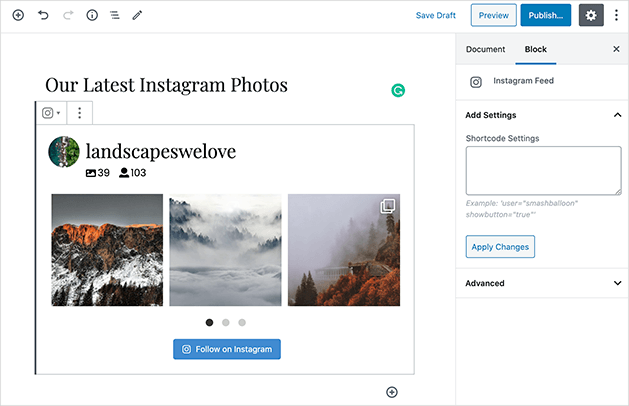This image depicts a user interface of a website management application. The interface features a clean, white background. At the top, there is a thin, grayish navigation bar, approximately an inch thick, adorned with several icons. On the top left corner, there is a plus symbol followed by back and forward arrows, an information button, a tabs button, and an edit button. To the right within the navigation bar, there are buttons labeled "Save Draft," "Preview," "Publish," and "Settings."

Below this navigation bar, on the left side of the interface, there is a section that resembles an Instagram post. The section is headed with the text "Our Latest Instagram Post" and is accompanied by a green refresh button. The Instagram post preview includes the caption "Landscapes we love," along with three images, a blue "Follow on Instagram" button, and additional details indicating 39 images and 103 next to a user icon.

Adjacent to this Instagram section, on the right side of the interface, there are various settings options for managing the post. These options include buttons for "Document" and "Block," settings for "Shortcode," and an "Apply Changes" button. There is also an "Advanced" tab available for more detailed configurations.